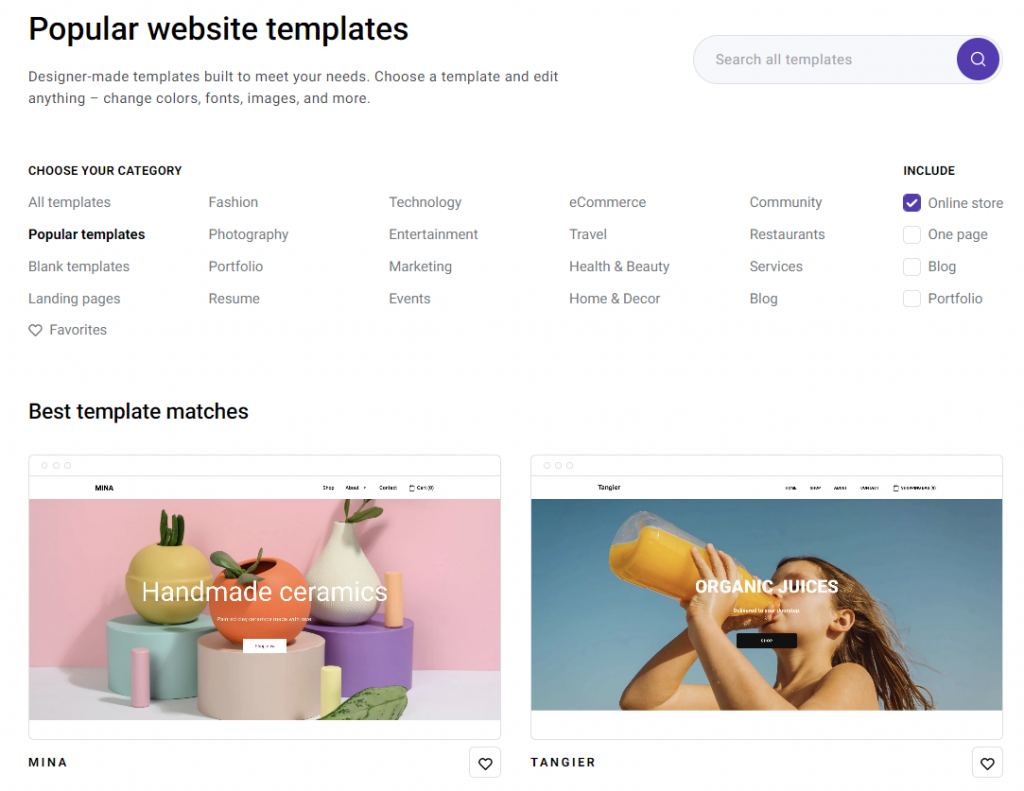This image features a website builder interface, potentially from a platform like Wix, displayed on a clean, white background. In the top left corner, the interface highlights "Popular Website Templates," with a description underneath stating, "Designer-made templates built to meet your needs. Choose a template and edit anything: change colors, fonts, images, and more." To the right, a search box with a purple search icon invites users to "Search all templates."

Below the search box, users are prompted to "Choose your category," which includes various options. The categories listed are:
- All templates
- Fashion
- Technology
- E-commerce
- Community
- Online Store (checked)

Additionally, there are several other template categories listed in sections. The "Popular Templates" section includes:
- Photography
- Entertainment
- Travel
- Restaurant
- One-page
- Blog
- Portfolio

The "Blank Templates" section includes:
- Portfolio
- Marketing
- Health and Beauty
- Services
- Landscape
- Landing Pages
- Resume
- Events
- Home and Decor
- Blog

A heart icon is available for marking favorites.

Below the template categories, the interface showcases "Best Template Matches," featuring examples such as "Mina," which highlights handmade ceramics, and "Tangier," which depicts an orange juice template including an image of a child drinking juice from a large plastic container.